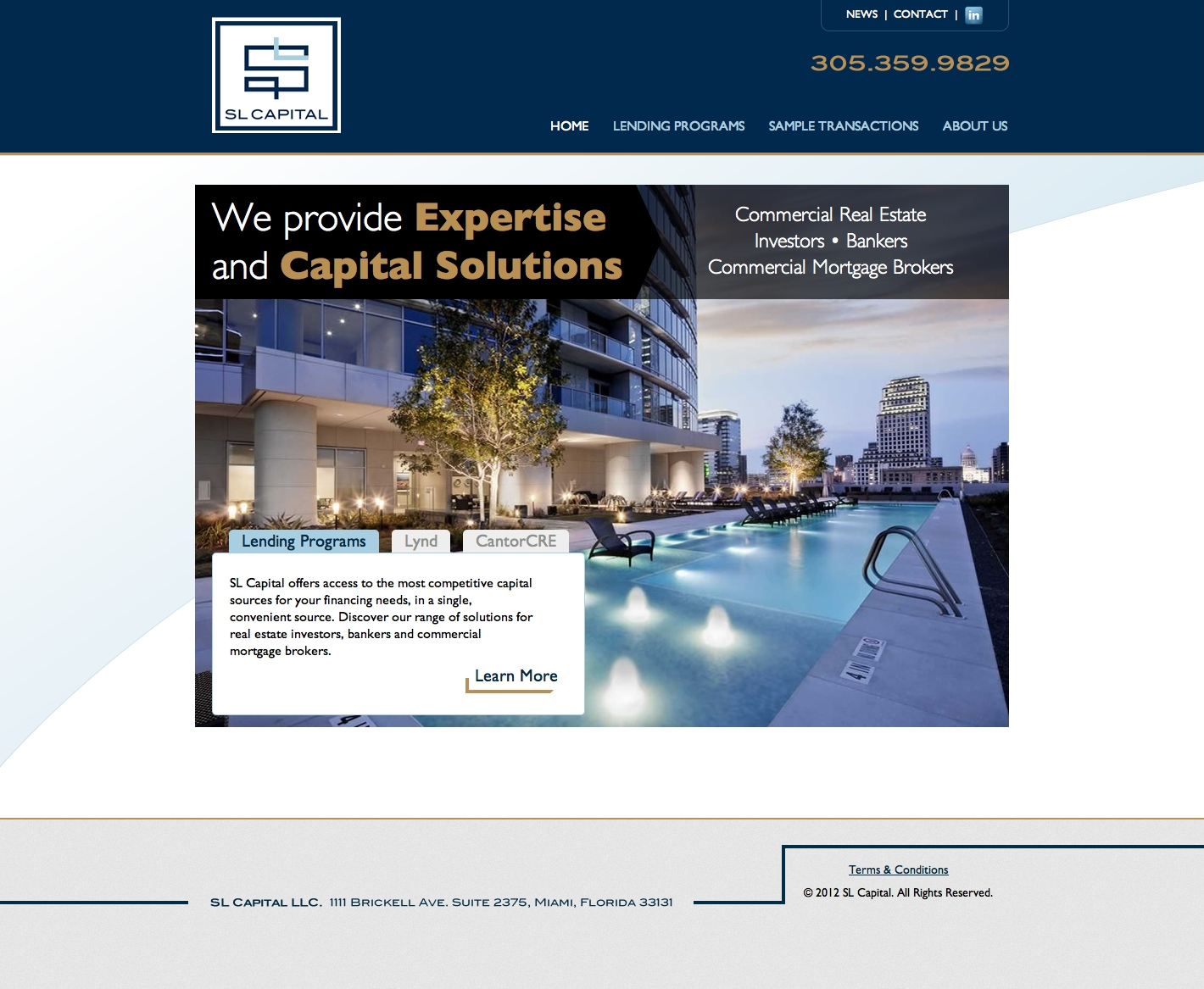Here is a detailed and cleaned-up caption for the image:

---

**SL Capital: A Premier Lending Program**

The image showcases the branding and interface of SL Capital, a sophisticated lending program. The logo prominently features a stylish "SL" with a snake-like "S" and a line at the bottom that curves and crosses to the left and down. This logo is set within a white box framed by a blue banner. Notably, the banner includes a "Home" tab in white text, along with links to sections such as Sample Transactions, About Us, and Lending Programs, all displayed in a light blue font.

Above these links, a large gold font displays the phone number: 305.359.9829. Additional links for News and Contact information, as well as a LinkedIn button, provide further navigation options. Centered prominently, a statement reads: "We provide expertise in capital solutions," written in gold. To the right, in white text, are target audiences such as commercial real estate investors, bankers, and commercial mortgage brokers.

The background features a stunning image of a condominium with an expansive view of a long, shallow pool equipped with in-water loungers. The scene is serene, dotted with trees and framed by towering buildings in the distance.

A box at the bottom of the image states: "SL Capital offers access to the most competitive capital sources for your financial needs." This box includes a "Learn More" button for further exploration. 

The Lending Programs tab, highlighted in blue, lists options such as "LYND" and "Cantor CRE." At the very bottom of the image, terms and conditions, copyright information, and the address—which is in Miami, Florida—are displayed in blue text.

---